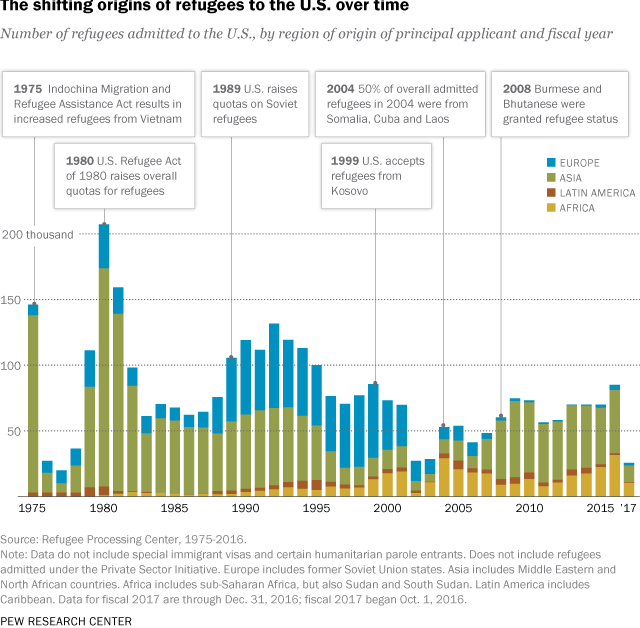This image is a detailed bar chart titled "The Shifting Origins of Refugees to the U.S. Over Time," illustrating refugee admissions to the United States from different regions between 1975 and 2017. The horizontal axis represents the years, while the vertical axis, ranging from 0 to 200,000, counts the number of refugees. The bars are divided into four colors, each indicating a region of origin: blue for Europe, green for Asia, red (rust) for Latin America, and yellow (desaturated gold) for Africa. Each bar segment signifies the number of refugees from these regions in a given year. Specific years are highlighted with annotations, such as 1999, when the U.S. accepted refugees from Kosovo. At the bottom of the graph, additional information and the source, Pew Research Center, are noted, suggesting this might be an informative piece from a textbook or news article.